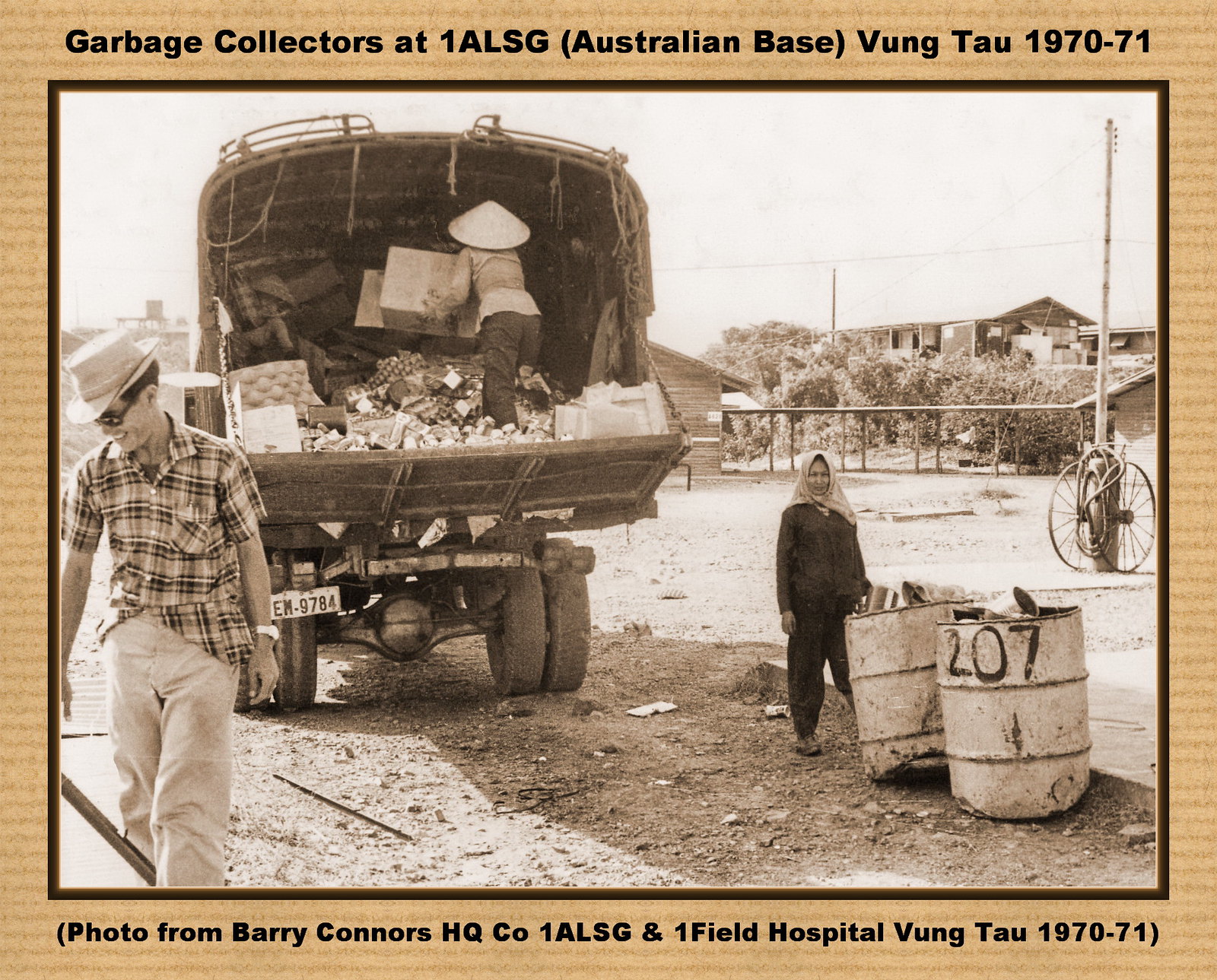This sepia-toned, vintage photograph from 1970-71, set within a light brownish-orange border with black lettering, captures a scene of Garbage Collection at the 1 ALSG, Australian Base in Vung Tau, Vietnam. The heading at the top of the image reads "Garbage Collectors," indicating the setting and timeframe, while the bottom credits the photograph to Barry Connors, HQ Co 1 ALSG, Onefield Hospital, Vung Tau, 1970-71.

In the foreground, a truck with an open back facing the viewer is central to the scene. A woman clad in traditional Vietnamese attire, including an Asian-style pointed hat, is seen dumping a box of garbage into the truck. To the left, a man in a straw hat, checkered plaid shirt, and white pants appears to supervise the activity, looking down as he stands nearby. Meanwhile, another woman, dressed in a dark shirt and trousers with a scarf on her head, is positioned next to two battered garbage containers. The background features a vast field dotted with tumbleweeds, faint outlines of buildings, and what appears to be wagon wheels on the far right. This photograph encapsulates a moment of daily life, framed beautifully with vintage photography and graphic design typography.